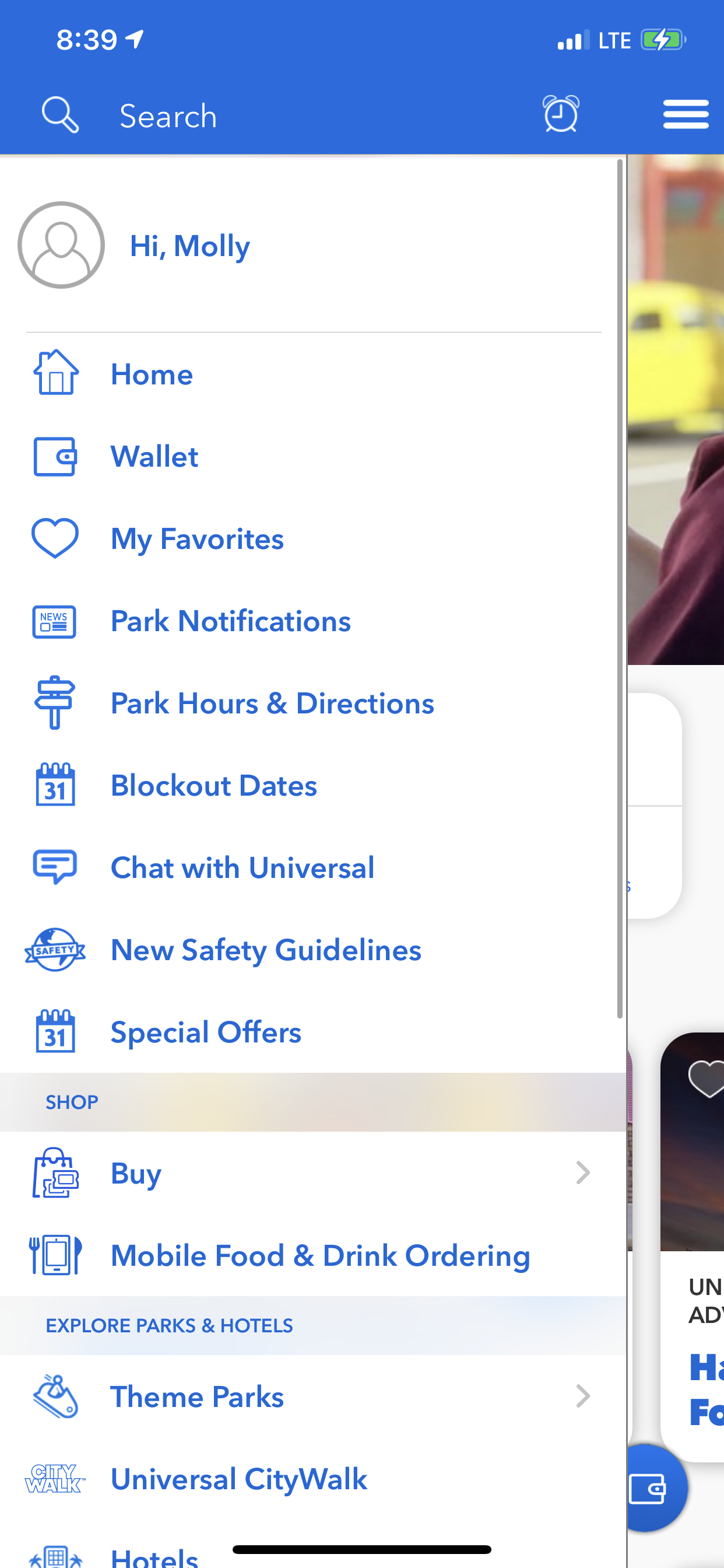A screenshot of a mobile application interface with a distinct layout. At the top of the screen, there is a white rectangle displaying a full battery icon at 83%, an alarm clock symbol, and a search bar accompanied by a hamburger menu icon to the right. Below this header, the user's profile name “Hi Molly” is prominently displayed. The main menu is organized into several sections, including Home, Wallet, My Favorites, Park Notifications, Park Home, Hours and Directions, Block Out Dates, Chat with Universal, New Safety Guidelines, and Special Offers.

Further down, there is a light gray rectangle containing options such as "Shop" accompanied by a right arrow, and "Mobile Food and Drink Ordering" suggesting convenience via mobile. There are also categorized sections to explore parks and hotels, featuring "Theme Parks," "Universal CityWalk," and Hotels," each indicated with a right arrow icon for easy navigation. 

Finally, at the bottom-middle of the screen lies a solid black bar, possibly serving as a navigation or action menu for quick access to other features or functions within the app.